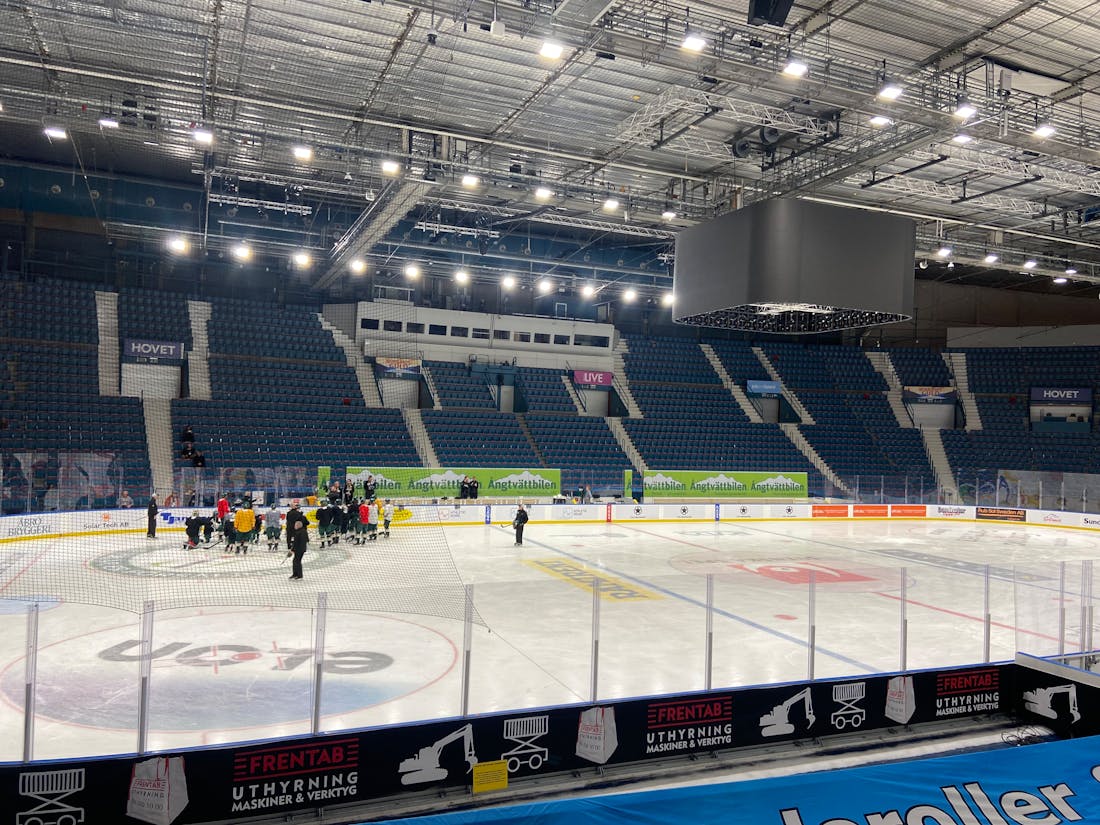The photograph captures a large, indoor ice hockey rink amidst an empty blue-seated stadium with an open-framed, industrial-looking ceiling adorned with floodlights. On the ice, a mixture of hockey players – donning yellow, red, black, and an occasional white uniform – are actively practicing, indicating it’s a training session rather than a match. The majority of the players are dressed in black, and they are supervised or perhaps coached by a few individuals standing further from the group. Clear plexiglass panels encircle the rink, serving as a barrier to protect spectators from stray hockey pucks. On the ice itself are various advertisements, including prominent logos for Elon and DeWalt. Additional advertisements and signs in green, orange, and some foreign languages can be seen scattered around the area, along with other distinctive markings such as the blue text reading " Rollers." The middle section of the stadium features a box seat area elevated above the regular seating. Overall, the rink is adorned with multiple colorful advertisements and designs, with the stark white ice serving as a backdrop to the vibrant practice session.